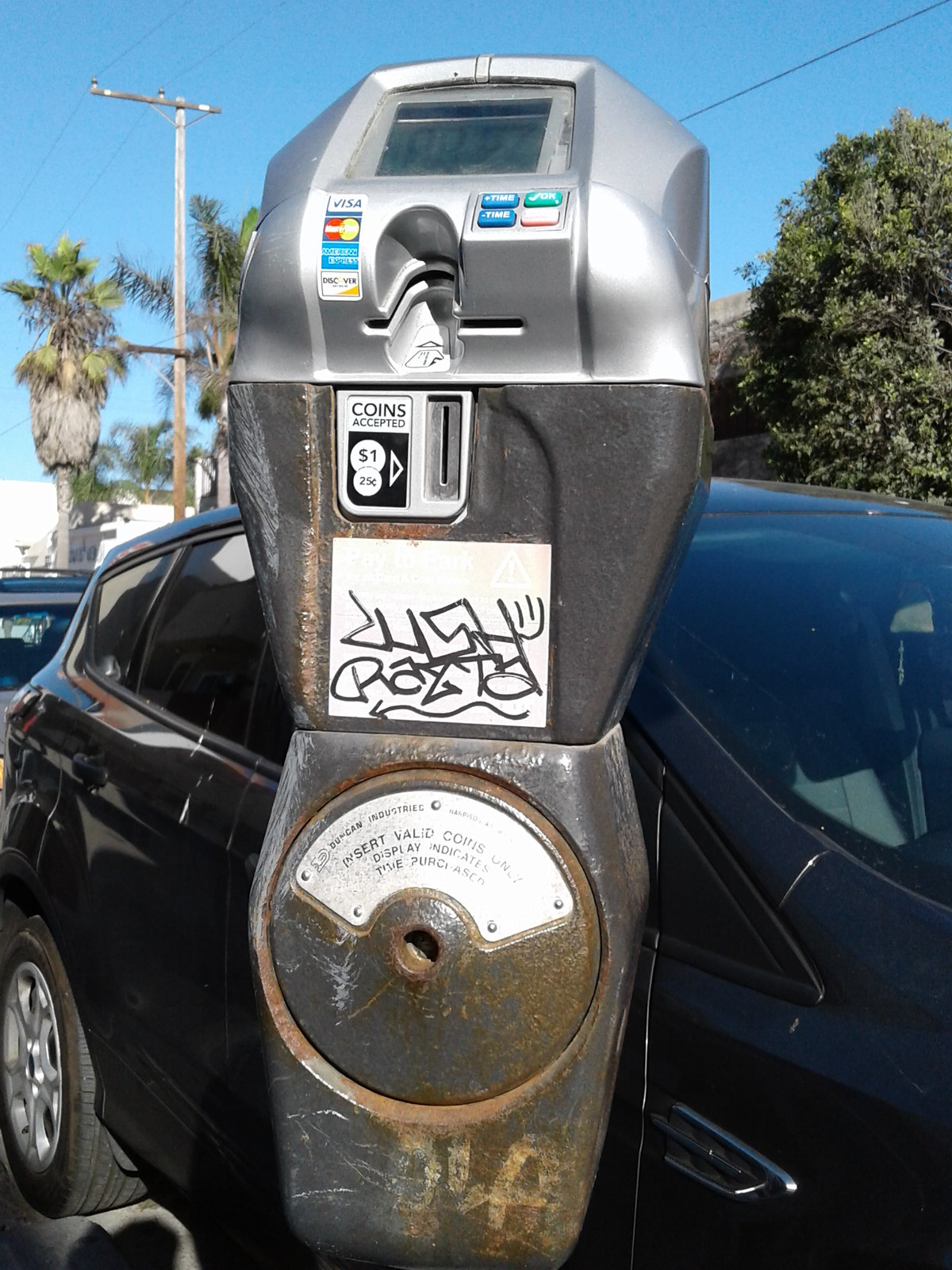This outdoor photograph features a close-up of a grey parking meter covered in unintelligible graffiti, particularly noticeable on the bottom half, which also has visible scratches. The top part of the meter appears newer and contains a display screen that is unreadable. The meter includes slots for both cards and coins, with stickers indicating it accepts Visa, MasterCard, American Express, and Discover, among other payment methods. The well-marked slots guide users on where to insert coins and cards. In the background, a black hatchback car with four doors is parked, with only one side visible. Beyond the car, there are two palm trees to the right of the meter, a power line, and a larger tree providing additional scenery. The sky above is light blue and clear, enhancing the outdoor setting.